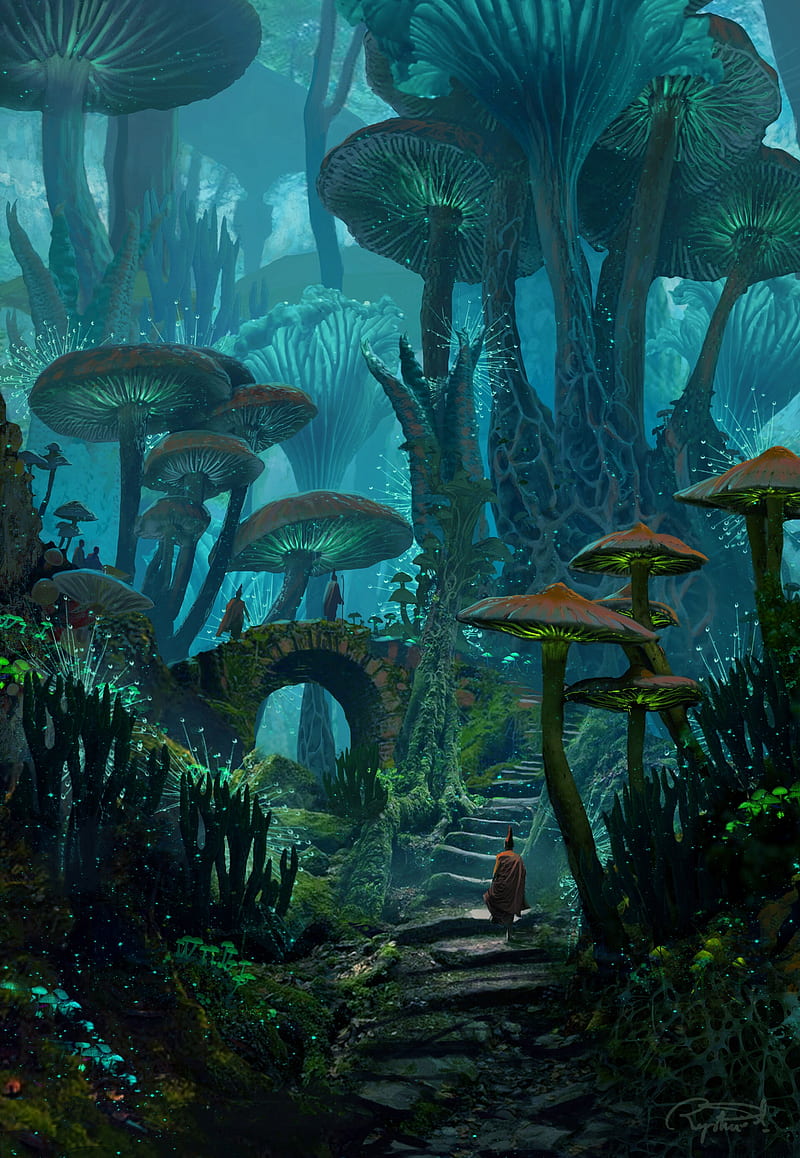The image depicts a fantastical, otherworldly landscape dominated by towering mushrooms that reach heights of 30 to 40 feet. The scene is set under a murky, obscured sky, completely hidden by the expansive mushroom caps that cast a surreal glow in green and blue hues, illuminating the environment. A stone staircase leads up to the base of these immense fungi, where a lone figure, possibly a human dressed in monk-like attire, is seen walking. Below, a stone bridge spans a small valley, with two more figures crossing it towards the towering mushroom patch. The scene hints at a possible meeting place beneath or behind the giant mushroom cluster, shrouded in mystery. This digital artwork, with its strange and foreign flora, conjures an ambiance of a distant alien world.